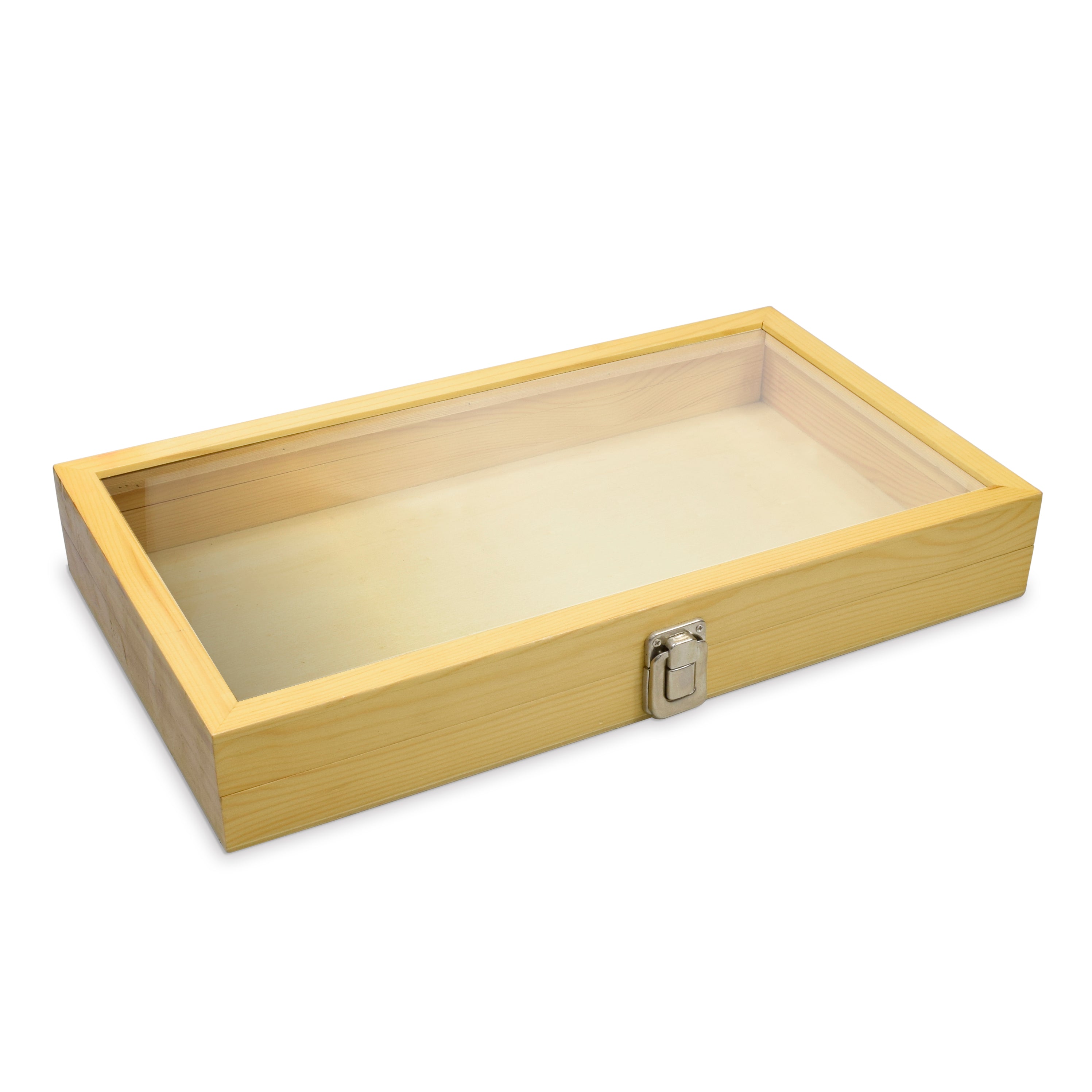The image showcases a wooden display box with a light yellowish hue, possibly made from maple or pine wood, giving it a natural and unfinished appearance. The box, measuring approximately 24 inches long, 16 inches wide, and about 6 inches tall, features a clear plexiglass top that allows visibility of the contents inside. The top is secured with a chrome-colored metal latch, reminiscent of suitcase clasps, which firmly holds the box closed but does not lock. Positioned on a white background, the box casts subtle shadows on the left side and front, creating a slightly slanted perspective where the left side angles towards the bottom left of the image, and the right side angles towards the top right. The interior sides match the wooden exterior, while the bottom appears to have a lighter, possibly white shade. Overall, the image provides a detailed view of the box, highlighting its construction and the see-through nature of its plexiglass top.